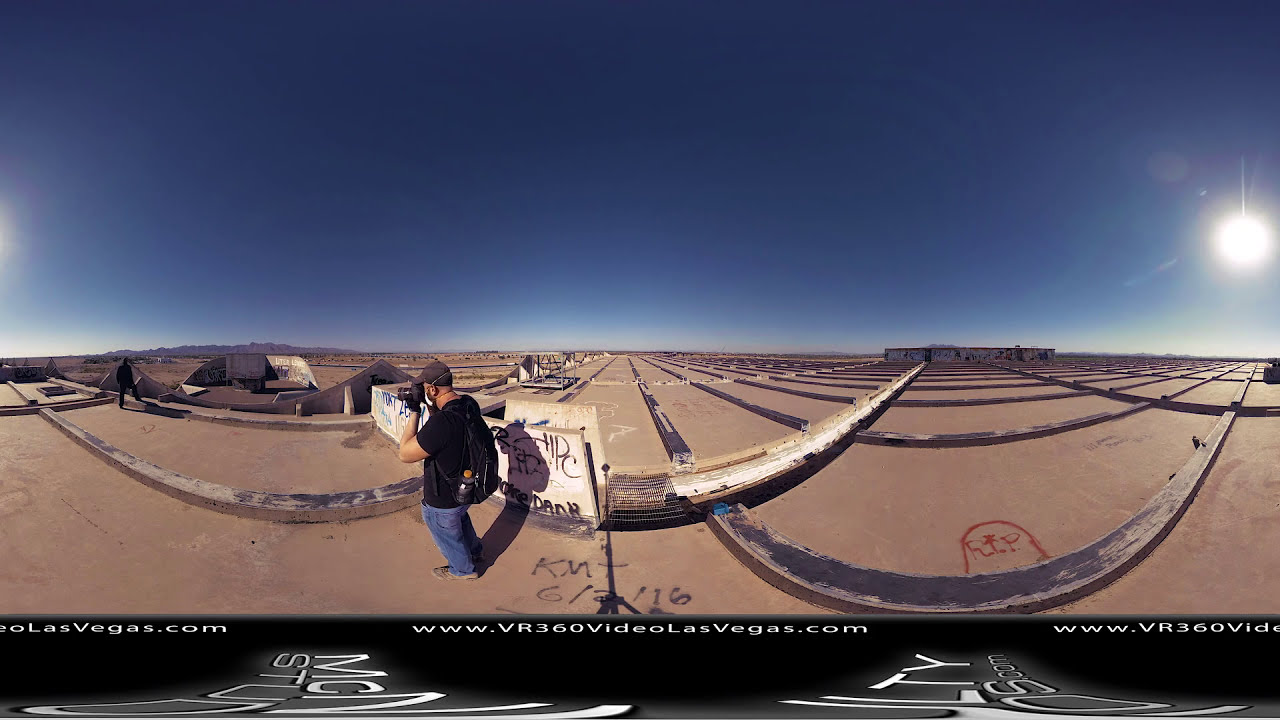The wide-angle photograph captured during a clear sunny day in a desert area features a distorted view where straight lines appear bent. Dominating the left side, a man facing left holds a black camera with a long lens up to his head. He wears a gray cap, black t-shirt, blue jeans, brown shoes, and a black backpack. Behind him, graffiti on the ground reads "KMT" with "612116" underneath. Further right, additional graffiti depicts a red headstone inscribed with "RIP." Parallel tracks start from the back and curve around, with one extending from a building in the background, leading to the foreground near some plywood adorned with white and more graffiti. A black line with a website address, "www.vr360videolasvegas.com," runs across the bottom. The upper right corner highlights the bright sun encircled by a yellow ring set against a dark blue sky, transitioning to a lighter blue at the bottom.